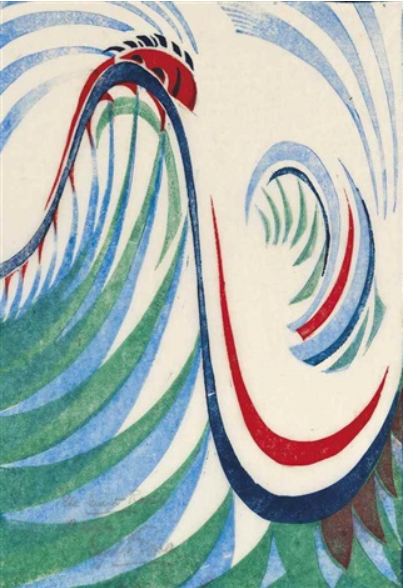In this abstract painting set against a white, textured background, a striking blue line dominates the composition. This line starts from the middle left, rises in a waveform, dips dramatically, and then ascends again towards the right. Along its path, it is accentuated by a red line that arcs above it, particularly highlighting the dip. Beneath this blue line, undulating, curving green spikes, shaded with blue, reach up towards it, creating a dynamic interplay of colors and shapes.

The artwork also features several blue arches in both top corners, thicker on their left sides and tapering to points on the right. Additional elements include more blue, red, and green curved lines in the middle, some forming a C pattern above the lower part of the main blue curve. Notably, a red and black shape, resembling a ladybug, is positioned at the top left corner near the blue arches.

The left side of the painting showcases various green and blue strokes, resembling grass blades, with hints of brown in the bottom right corner. These strokes provide the largest and most vibrant splashes of color. The overall composition is a chaotic yet harmonious blend of flowing lines and vivid colors, creating a dynamic visual experience.